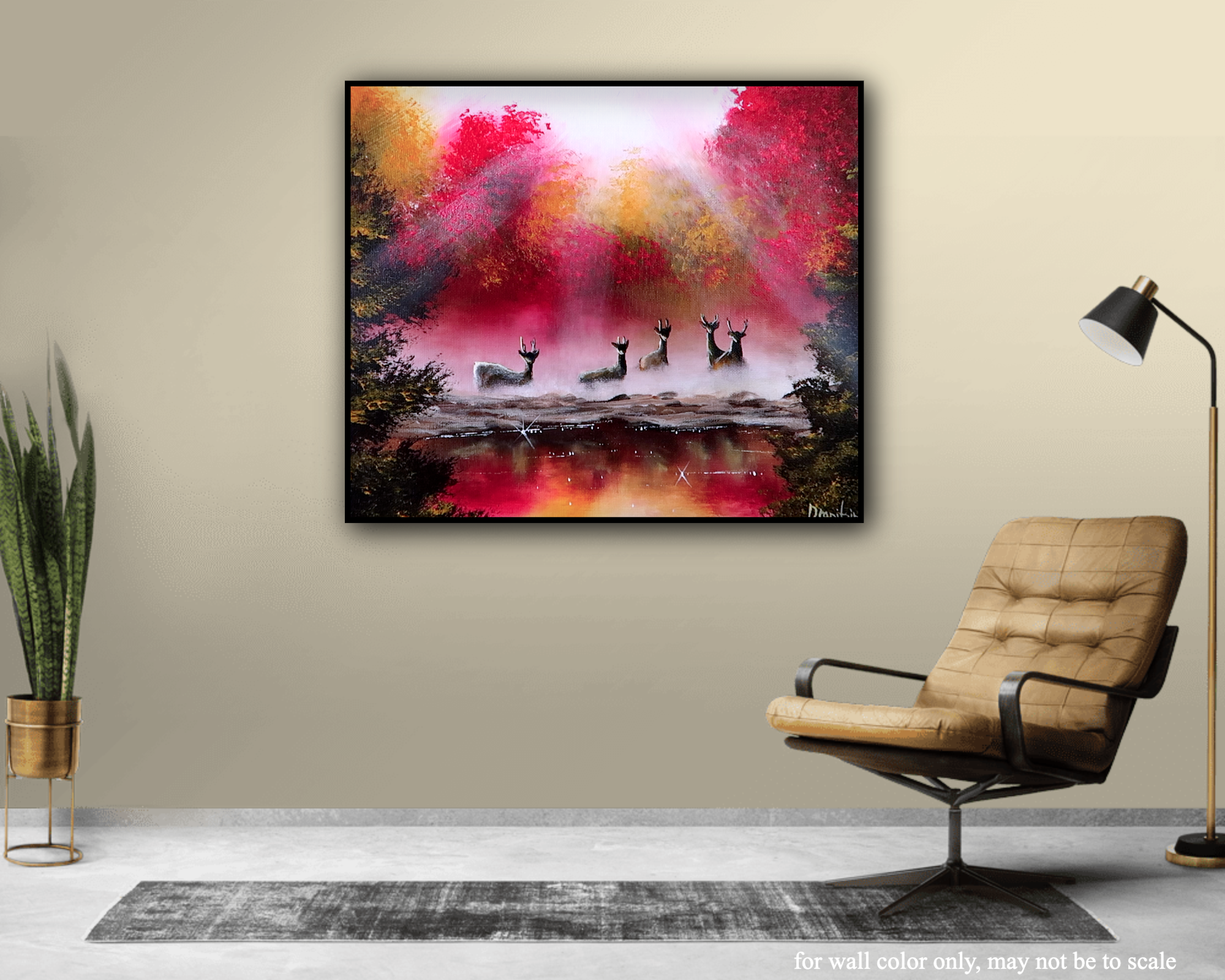The image depicts a sparsely furnished indoor setting, which could be an office or waiting room. The room features a beige wall adorned with a striking painting at its center. The painting showcases a serene outdoor scene with five deer standing amidst the mist on a rocky ground, surrounded by autumn trees in vivid shades of red, orange, and yellow. Rays of sunlight stream through the trees, adding a sense of depth and natural beauty to the artwork. To the very right of the image is a slightly reclined, light brown leather office chair with black armrests, accompanied by a silver and black standing lamp positioned behind it. On the left, a green variegated snake plant sits in a golden pot, adding a touch of greenery to the space. The floor consists of a grey-white granite surface with a darker grey weathered runner stretching horizontally. Overall, the painting serves as the main focal point, bringing vibrant color and nature into an otherwise muted room.